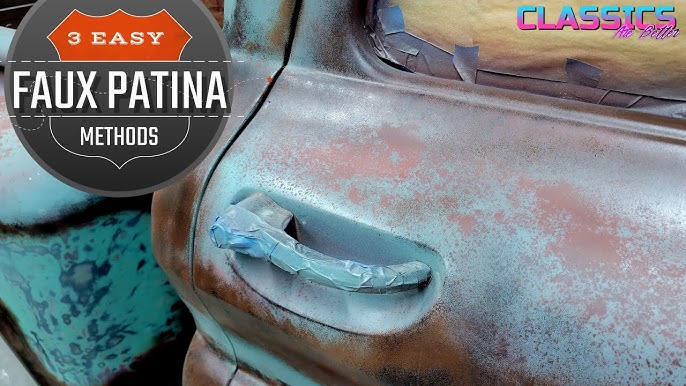The image is a close-up color photograph of a very rusty car door, prominently displaying a heavily corroded and taped-over door handle. There is a distinct blue-patina effect on the door, giving the appearance of rusted blue paint. The car window is covered with brown paper from the inside, secured with blue masking tape which also exhibits the same rusty blue paint effect. In the top left corner of the image, there is a black circular graphic with a red-tinted top, resembling a shield or highway sign, containing white text that reads "Faux Patina," with smaller text below stating "Three Easy Methods." In the top right corner, partially obscured pink and blue lettering reads "Classics are better."